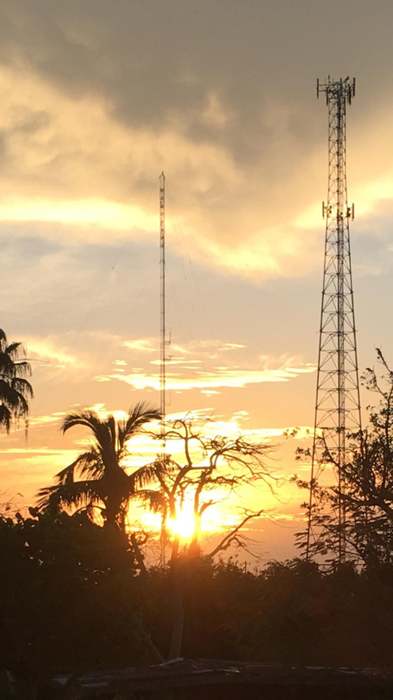This is a detailed vertical rectangular photograph capturing a serene landscape during sunset. The picture is divided into three main sections: the sky at the top, the water in the middle, and land with trees at the bottom. The sky is adorned with an array of clouds, blending shades of light and dark gray, tinged with vibrant orange and yellow hues near the horizon. As the eye moves down, traces of blue mix with the gray and yellow, signifying the approaching twilight. Prominently on the right side of the image stands a tall metallic tower, likely a cell phone or radio tower, with a slender metal structure visible in the distant background. The middle section of the photograph showcases the sun setting over a body of water, casting a shimmering reflection. The bottom part of the image is dark, dominated by the silhouettes of trees, including distinctive palm trees. This composition highlights the serene transition of the day, framing the metallic structures against the captivating sky and tranquil water, all grounded by the shadowed tree line.